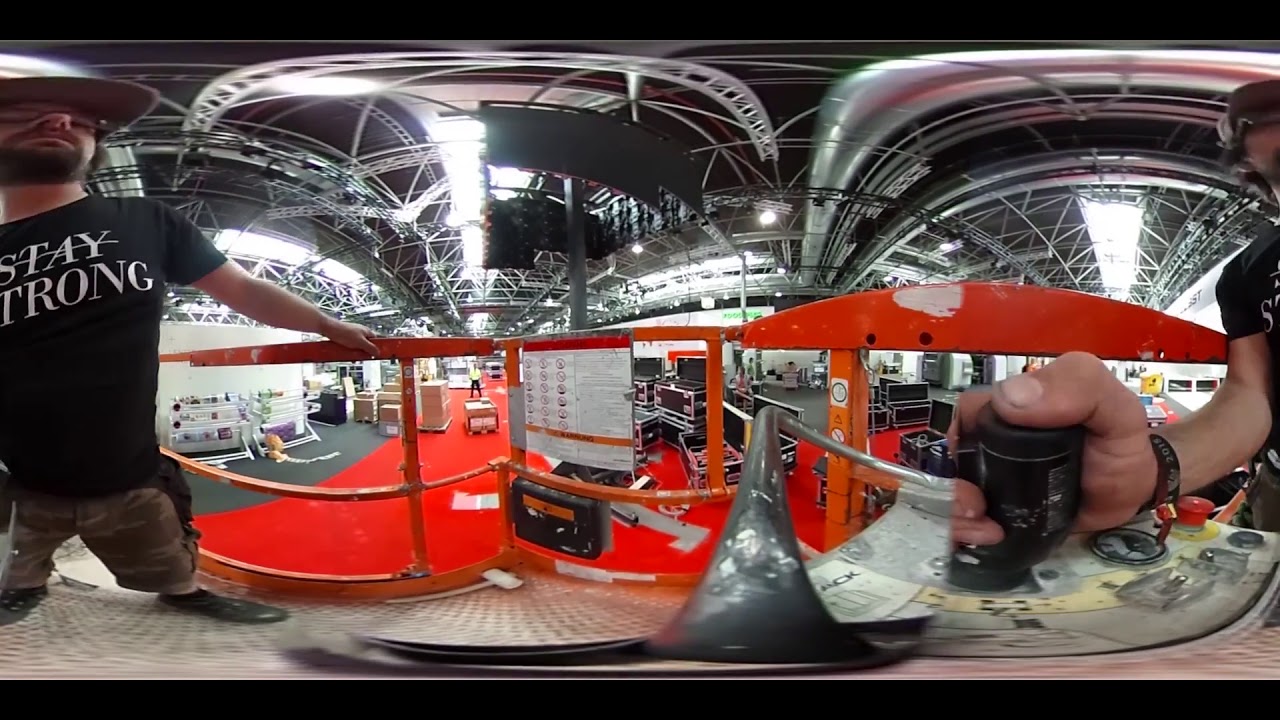In this photo with thin black lines at the top and bottom, creating a convex distortion, we see a scene from a bustling warehouse or factory floor. On the left, a young man with a neatly trimmed black beard and a hat is wearing a black short-sleeved t-shirt with white text saying "Stay Strong," where the word "Stay" has a line through it. He also has on grey shorts and grey shoes. Behind him, the ceiling is crisscrossed with metal rafters, pipes, and large fluorescent lights illuminating the space. There are stacks of cardboard and black freight boxes, along with machinery and several workers engaged in their tasks. On the right side of the image is another man who could be a mirror-flipped version of the first. This man has his hand on a black cylindrical handle, likely part of a crane or lift mechanism, and wears a black watch on his right wrist. The two men are standing on an elevated metal platform with an orange railing, hinting at industrial safety protocols. The overall image feels as though it has been viewed through a pair of safety goggles, adding to the industrial ambiance.